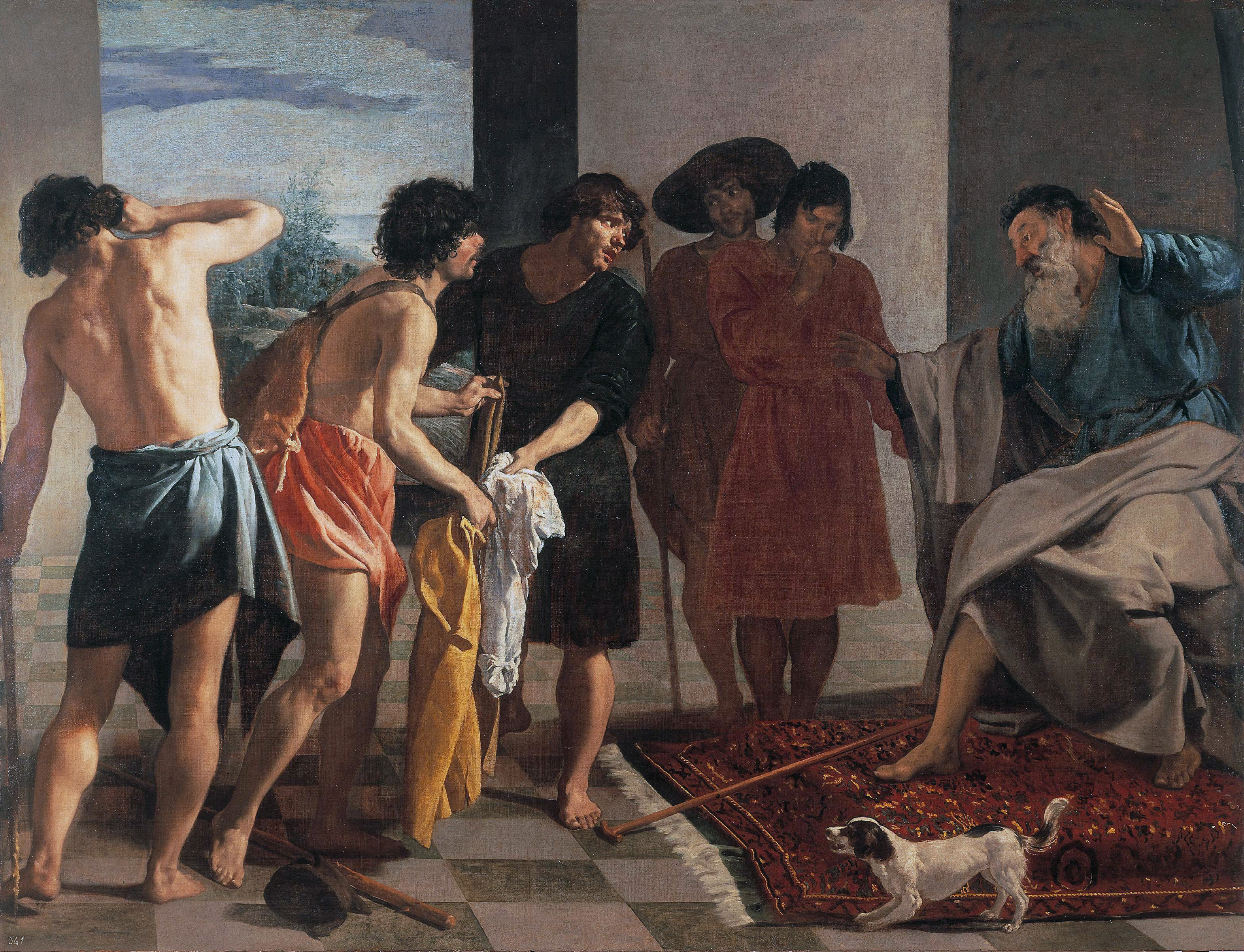The painting captures a classical, possibly neoclassical, scene set in an ancient European, likely Italian, context. The central focus is an older man with a heavy white beard and dark hair, dressed in blue and gray robes. His hands are outstretched, possibly in a gesture of pleading or commanding "stop," and he appears to be falling backward onto an ornate Turkish rug with white fringe on its right side. Surrounding him are five younger men, likely students, dressed in various robes and tunics.

On the left side, two barefoot figures gaze towards the falling man, while in the center, another man in peach-colored robes looks down with his hand near his nose. This man, assumed to be the opponent in the struggle, stands near a dropped cane, suggesting a recent altercation. Next to him, a man wearing a large-brimmed hat and a black robe stands in contrast to another figure adorned with a simple blue cloth around his waist.

The scene takes place on a checkerboard floor with light and dark gray tiles, adding depth to the composition. The backdrop features black and gray walls with an opening that reveals elements of nature—trees, water, and sky—suggesting a serene environment outside. Finally, a small black and white dog, seemingly barking, is positioned near the rectangle rug, adding an additional layer of liveliness to the intricate scene.